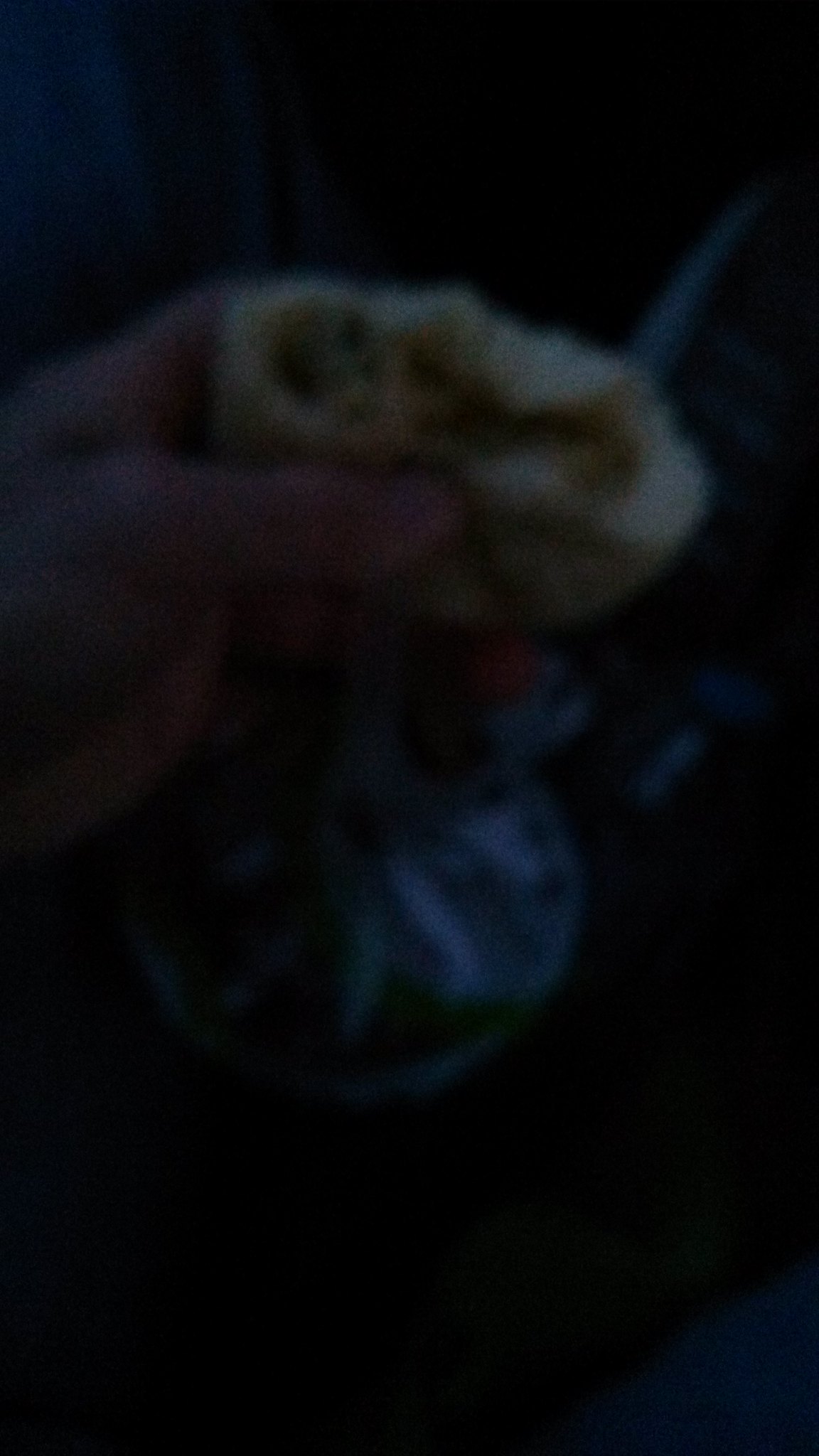The image portrays a dark, blurry, and unfocused scene, primarily set against a black or near-black background, possibly indicating a nighttime or early morning setting. Centrally, a white Caucasian individual's left hand is visible, holding a partially bitten food item. The bitten section reveals an interior that might contain cheese and meat, suggesting it could be a burrito or a sandwich. There is also mention of a glass with a round base and stem, likely positioned beside or behind the hand, and another potential glass in the backdrop. A small blue object or flash of color is present near the lower part of the image, alongside a plastic bag. The overall image is vertical in orientation, with the unclear white and blue objects occupying about half of the visual space.